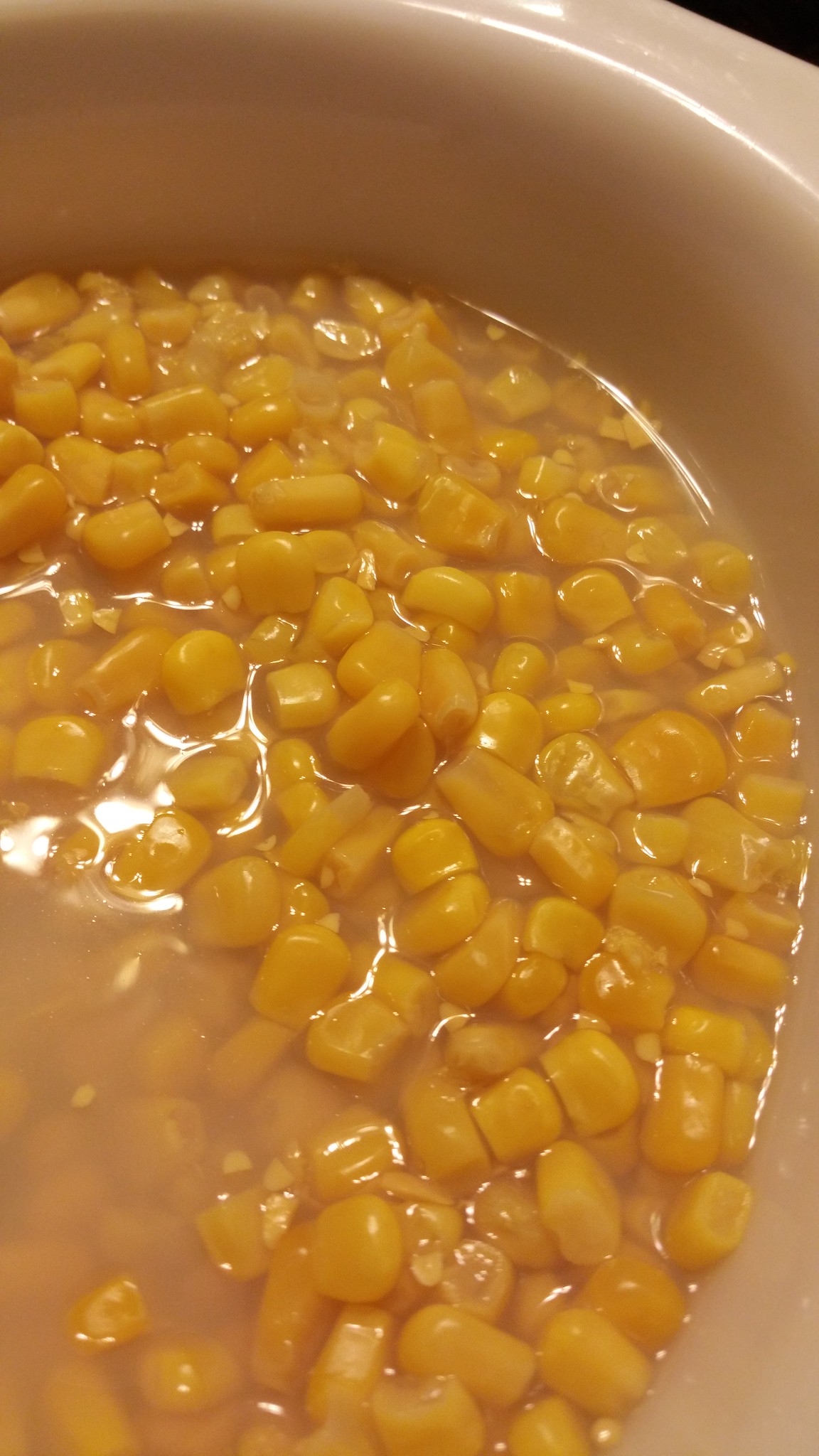This is a vertical color photograph featuring a cream-colored, or potentially pinkish beige, ceramic bowl, partially cropped and only showing the top right portion. The bowl is filled about halfway with bright yellow corn kernels floating in the cloudy liquid typical of canned corn. The kernels, over a hundred in number, are primarily concentrated towards the upper right of the frame, while the lower left shows more of the liquid. The photograph has a minimalistic composition, showcasing just the bowl and the corn with no visible background, hinting that it may have been purposefully framed or cropped this way. The absence of any additional ingredients or seasoning suggests that the corn was simply dumped from the can, creating an unadorned but intriguing visual depiction.